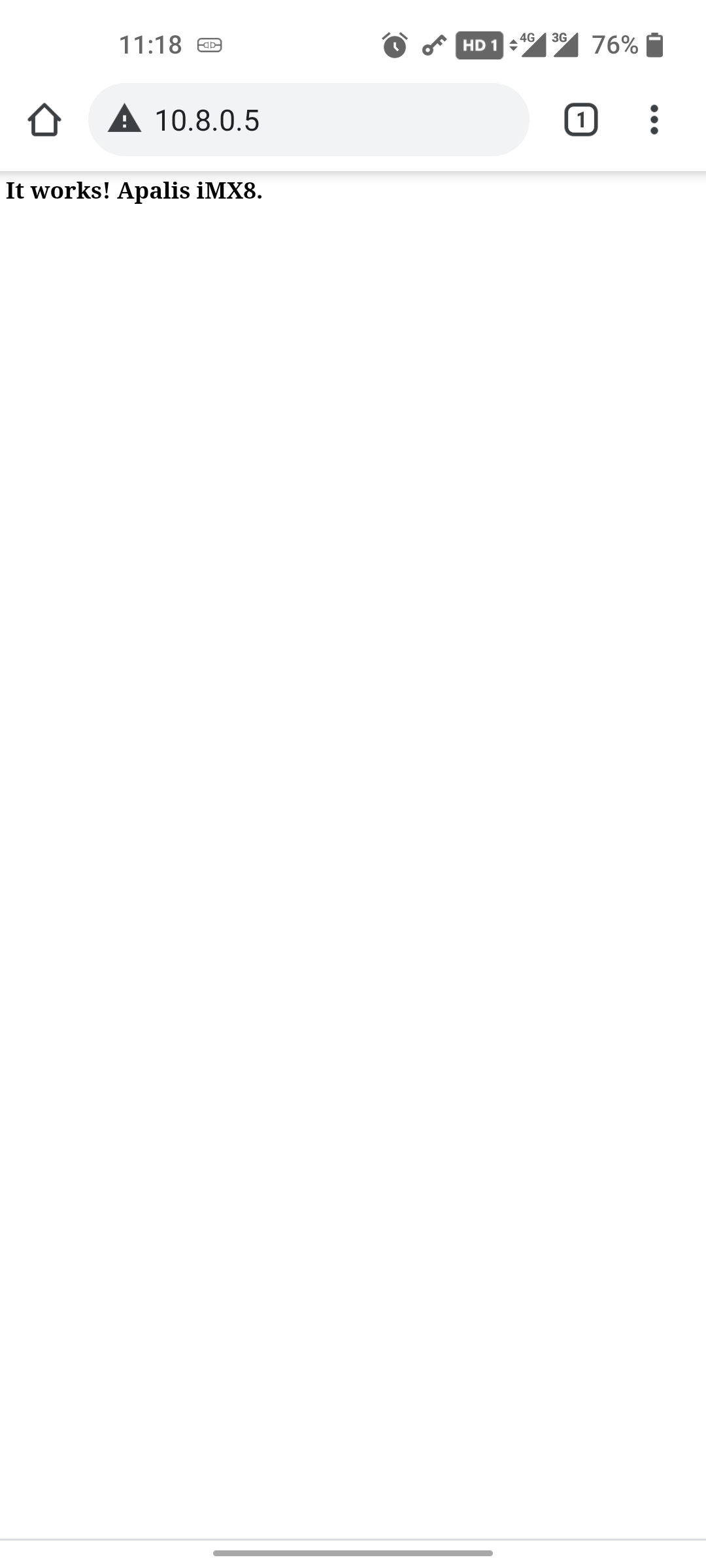Screenshot Description:

At the top of the screenshot, the status bar displays the current time, 11:18, on the left side. Next to the time, there is an oval-shaped icon whose function is unclear, followed by a clock alarm icon, and another icon resembling a key. Following these, there is an icon labeled "HD1," which may indicate an HD call or network mode. The status bar also shows two signal bars, which could imply the phone supports dual SIM functionality. 

Further along, the battery percentage is indicated as 76%, accompanied by a standard battery icon. Moving to the right edge of the status bar, a home icon is visible, designed as a combination of a triangle and a square. Below the status bar, a caution triangle with an exclamation mark inside displays. Right next to this symbol, the number 10.8.0.5 is prominently displayed. 

Further details include a small square icon with the number "1" inside it and three vertical dots, suggesting menu options. Below these icons, there is a text that reads, "it works, upholds I-M-X-S." The rest of the screen remains blank.